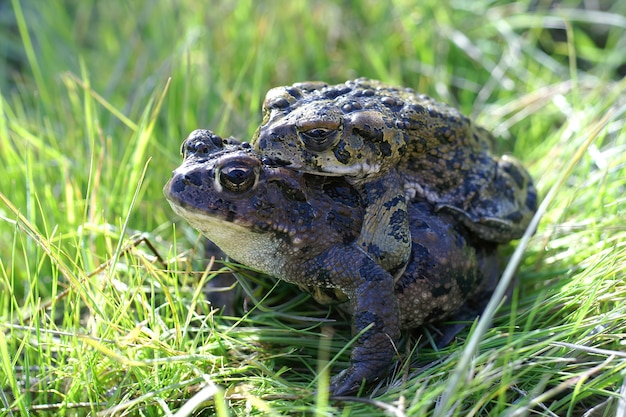This is a sharp, up-close daylight photograph capturing two toads in a lush, green, grassy area, indicative of spring or summer. The foreground grass is finely detailed, while the background is slightly blurred. The scene features a large, brown toad with a lighter-colored underside and black spots, facing to the left. This toad, which also has a white patch under its chin, is being mounted by a smaller, more green-colored toad, with similar black spots and characteristic bumpy skin. Both toads have their eyes open and appear to be relaxed, as if enjoying the day. The green-spotted toad on top seems to be hitching a ride, pressing down on the bushy grass beneath them. This image, with sunlight filtering through, beautifully captures the natural behavior and serene environment of these amphibians.